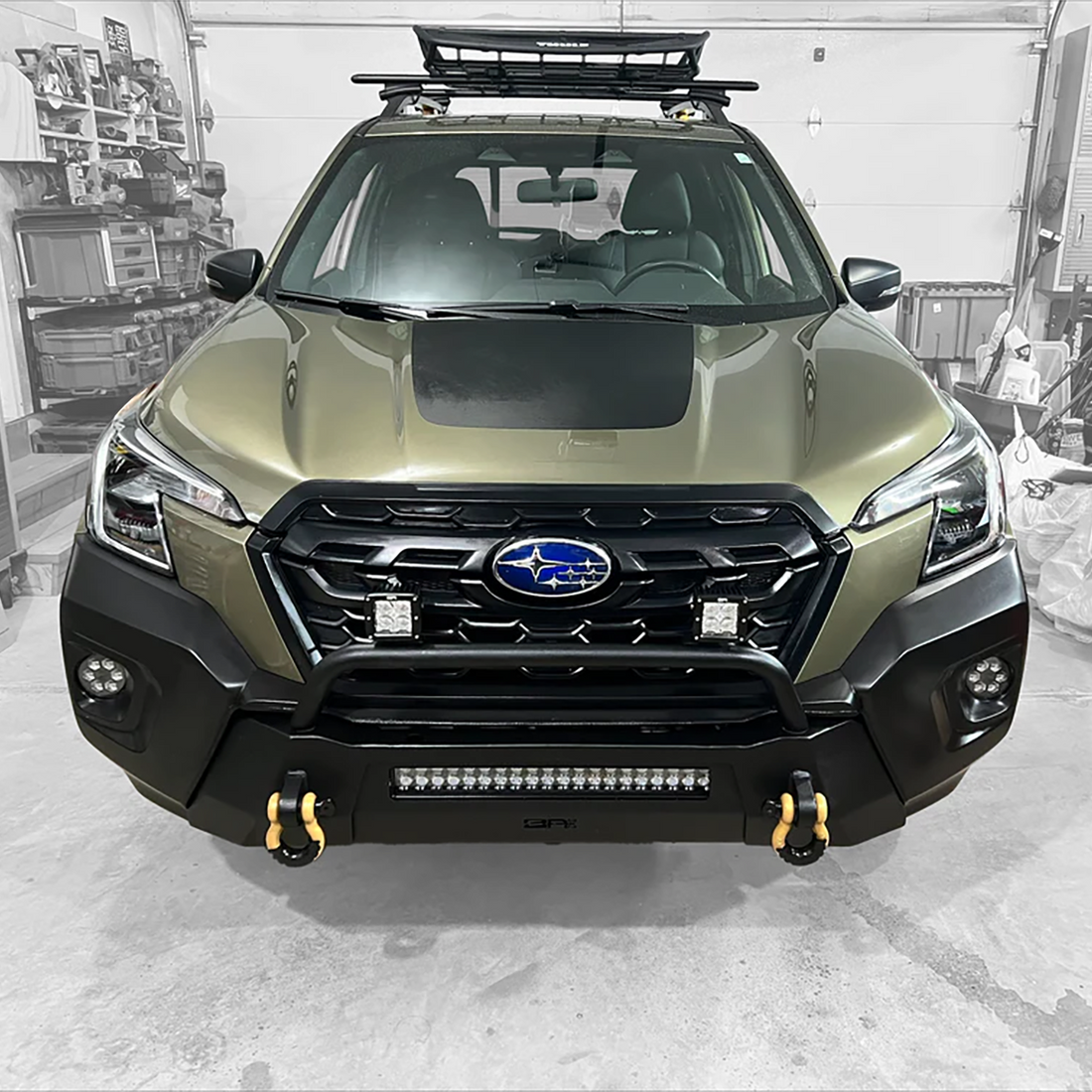This image captures the front view of a brand-new Subaru hatchback, meticulously showcased within a typical garage scene where selective coloring highlights the vehicle against a black-and-white backdrop. The Subaru, in a metallic olive green or sage hue, features a black panel on the hood. Prominently displayed is the Subaru's oval logo with a pattern of four-pointed star fins, set against a black grille and bumper equipped with a light bar and yellow tow hooks. The car sports roof and bike racks along with fog lights integrated into the bumper. Illuminated from above, the photo also reveals shadows beneath the car, which rests on a concrete floor. The garage’s closed door sits behind the car, surrounded by cluttered shelves and racks on the left, tools in the upper left corner, and miscellaneous items scattered on the right floor, creating a vivid contrast with the well-maintained vehicle.